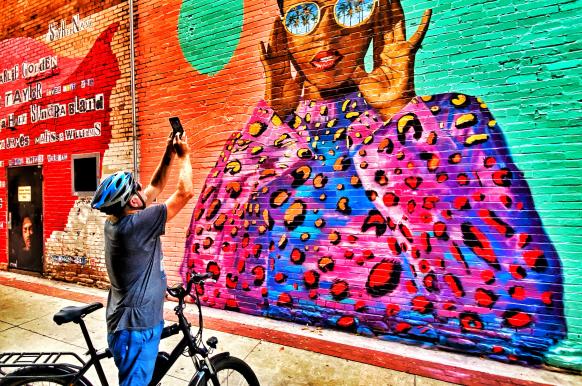A man is captured in this photo while riding his black bicycle, standing up from the saddle. He is dressed in denim jeans, a dark blue shirt, and a blue and black bike helmet. The man has his arms extended, holding a cell phone high above his head to take a picture of a vibrant mural on a wall in front of him. The mural features a dark-skinned woman adorned in a colorful sweater with shades of blue, purple, pink, and red, suggesting a cosmic theme. She wears oversized sunglasses that reflect palm trees, hinting at a tropical or Latin American setting. The background of the mural is split into bright orange and seafoam green sections, possibly including a green sun and some unreadable text on the far left. The woman's pose with her hands up to her ears contributes a sense of animated character to the artwork.